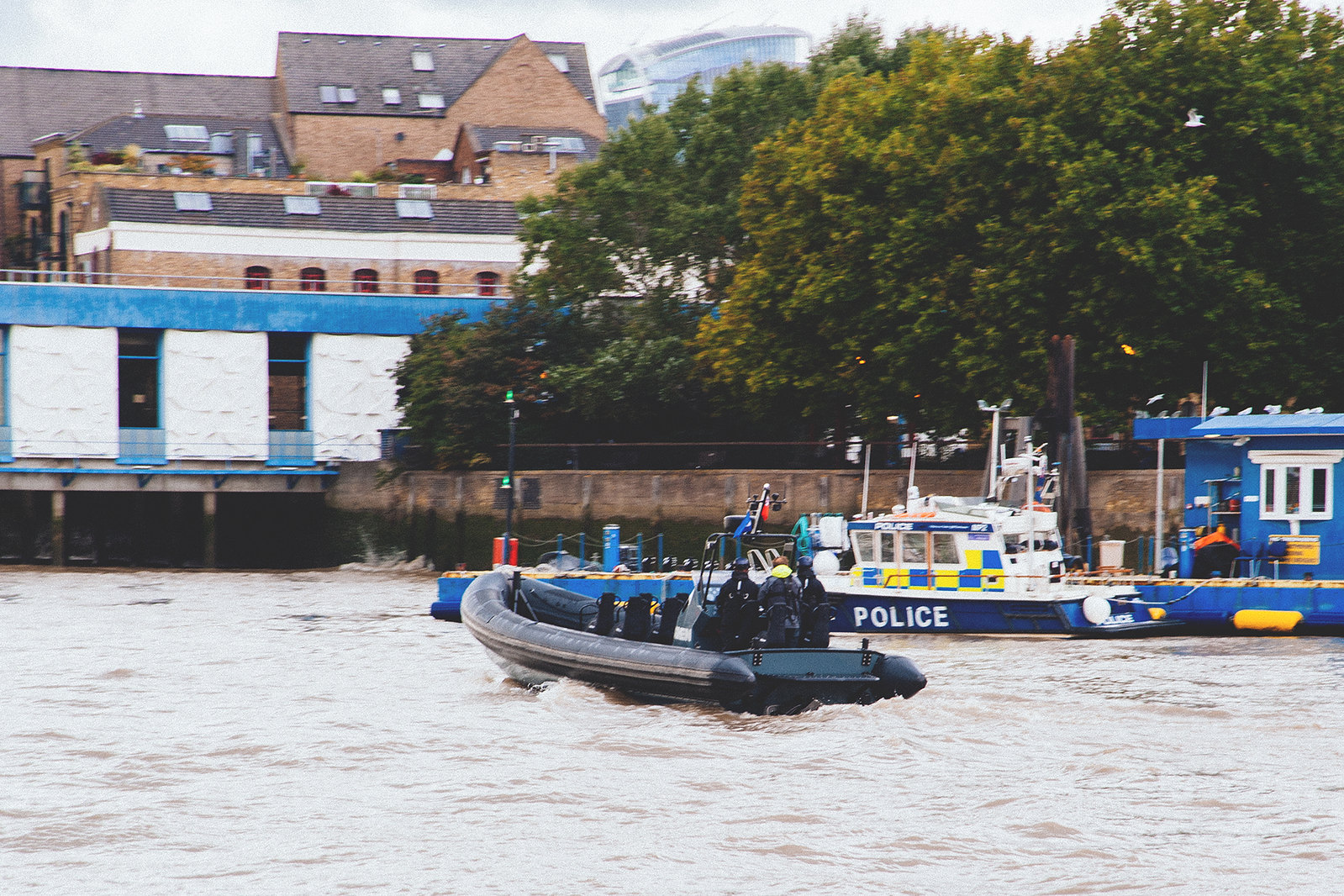The image captures a choppy body of water, likely a river in the United Kingdom or Europe, with two distinct boats. In the foreground, there's a black inflatable boat with several people in blue uniforms and various equipment onboard, suggesting it may be a military or special operations vessel. To its right, a blue and white boat marked "POLICE" with yellow and light blue checkered patterns is visible. In the background, a dock and pier can be seen alongside a concrete wall, several trees, and traditional brick buildings with dark brown tile roofs. A bridge spans the water, supporting a white building with a blue roof above. The sky is overcast, adding to the moody ambiance of the scene.